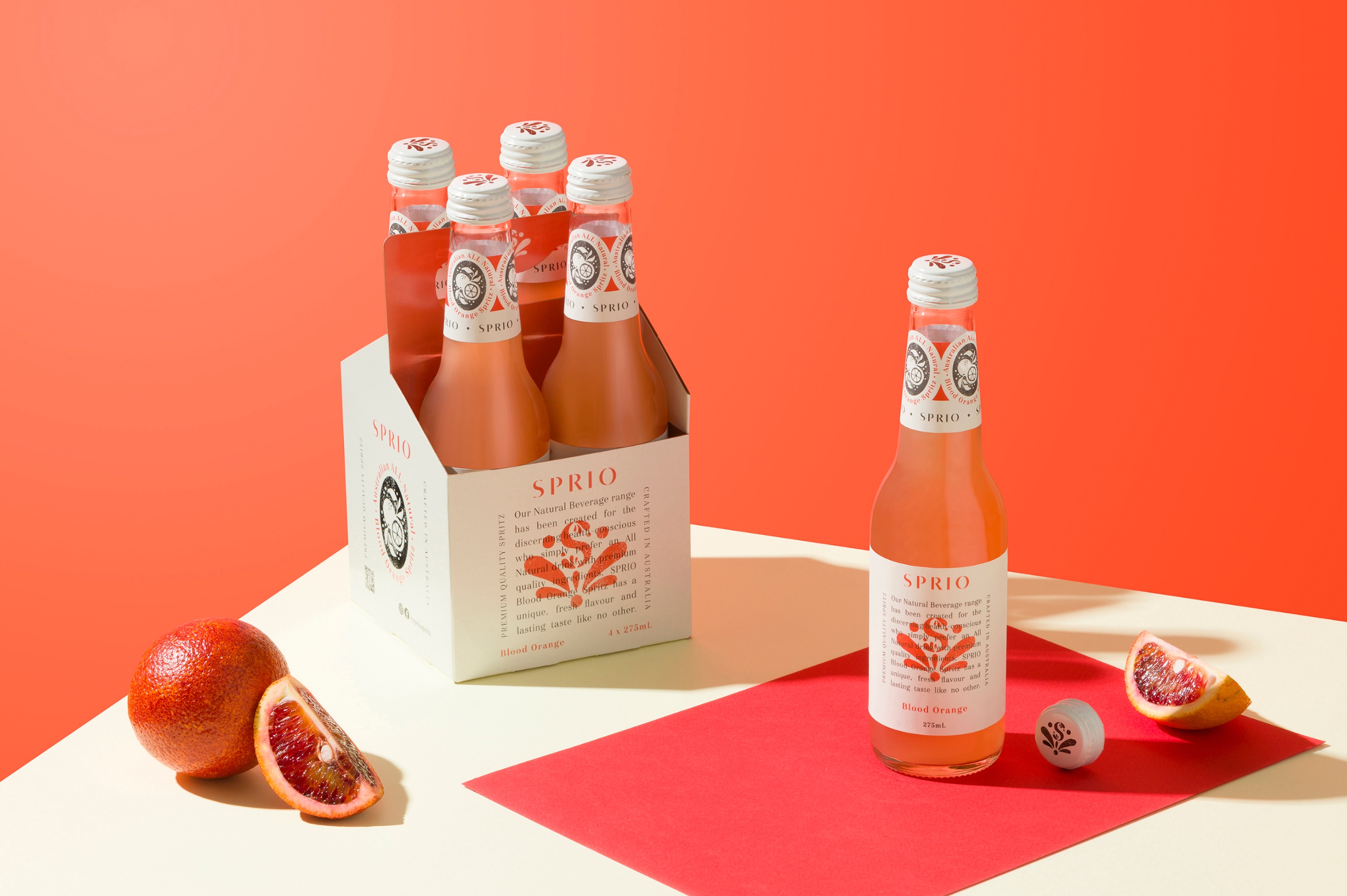The product image showcases a beautifully arranged four-pack of Sprio spritzers, featuring glass bottles with sleek white labels and matching white metal caps. In front of the four-pack sits an individual bottle on a vibrant red piece of fabric. The bottle's cap, displaying a leaf design, lies open on its side next to it. Adorning the white table are sliced segments of juicy blood oranges, enhancing the theme and flavor of the spritzer. The background of the image is a rich, dark orange color, creating a warm and inviting atmosphere that highlights the refreshing and citrusy essence of the Sprio blood orange spritzer.